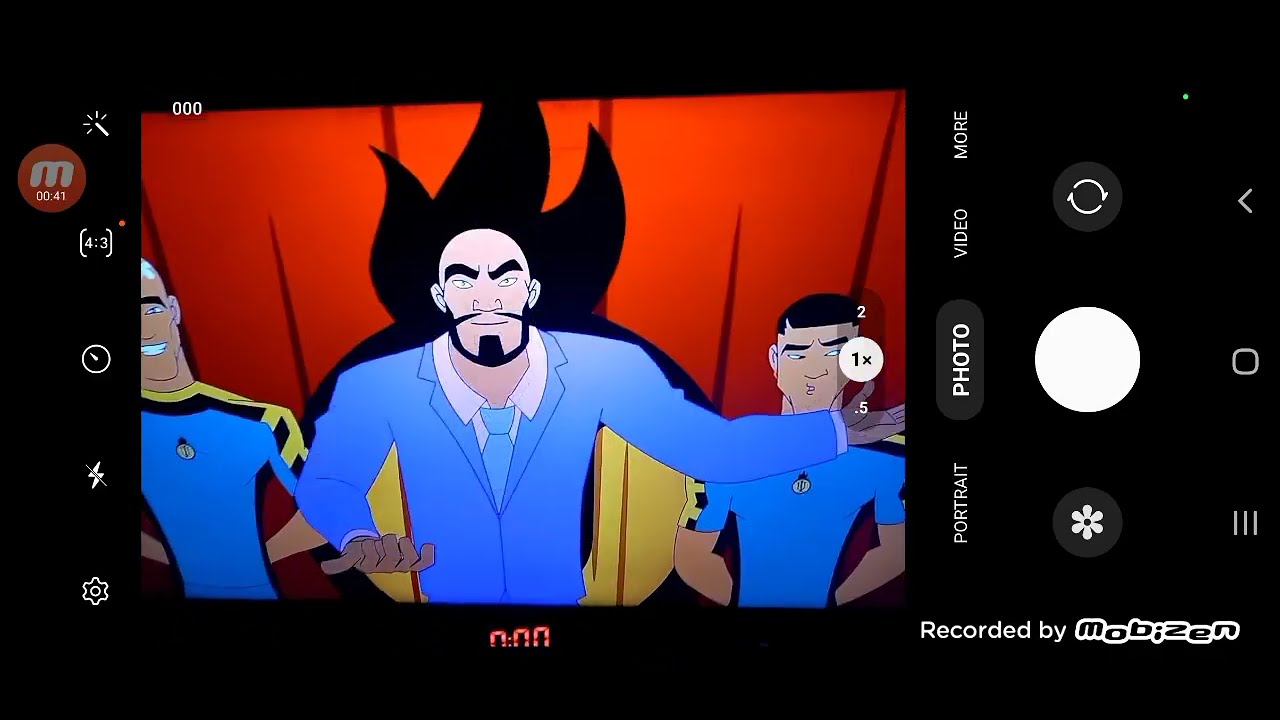This image appears to be a screenshot from a smartphone, depicting a cartoon scene involving three men dressed in Star Trek-like uniforms. The central figure is distinctly characterized by his bald head, heavy black eyebrows, goatee, and blue suit paired with a white shirt and blue tie. He exudes an ominous presence, emphasized by a shadowy or flame-like outline behind him and a red curtain backdrop. The two men flanking him are both wearing blue short-sleeve shirts. The man on the left has white hair and is smiling, while the man on the right has dark hair and is sneering. The smartphone screen features various app icons and controls, including buttons for "portrait," "photo," "video," and "more," situated on the left and right sides due to the image being flipped sideways. Additionally, there is a prominent white shutter button. At the bottom right, the image is marked with the text "recorded by Mobizen," and there are three "N" symbols below the central figure. The scene captures a distinctly animated and somewhat sinister tableau, framed by the typical interface elements of a mobile camera app.